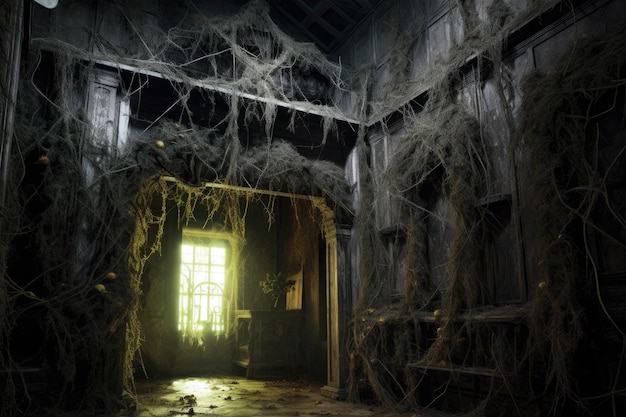The image depicts the eerie interior of an old, abandoned house with very tall ceilings, possibly around 20 feet high. This desolate space is shrouded in darkness, with walls painted in black or dark gray. The room is overtaken by thick cobwebs and hanging moss, covering the ceiling, door frames, and almost every corner, contributing to the overall spooky atmosphere. A muted, yellowish light streams through a window situated in the middle left section, casting an eerie glow that highlights the room's gloominess. The otherwise barren room features a solitary bookshelf or shelf near the window and gold door handles, barely visible through the layers of dust and neglect. The light from the window throws contrasting brightness in an otherwise gray and dark environment, emphasizing the dilapidated and forsaken state of the house, which resembles a setting straight out of a horror movie.